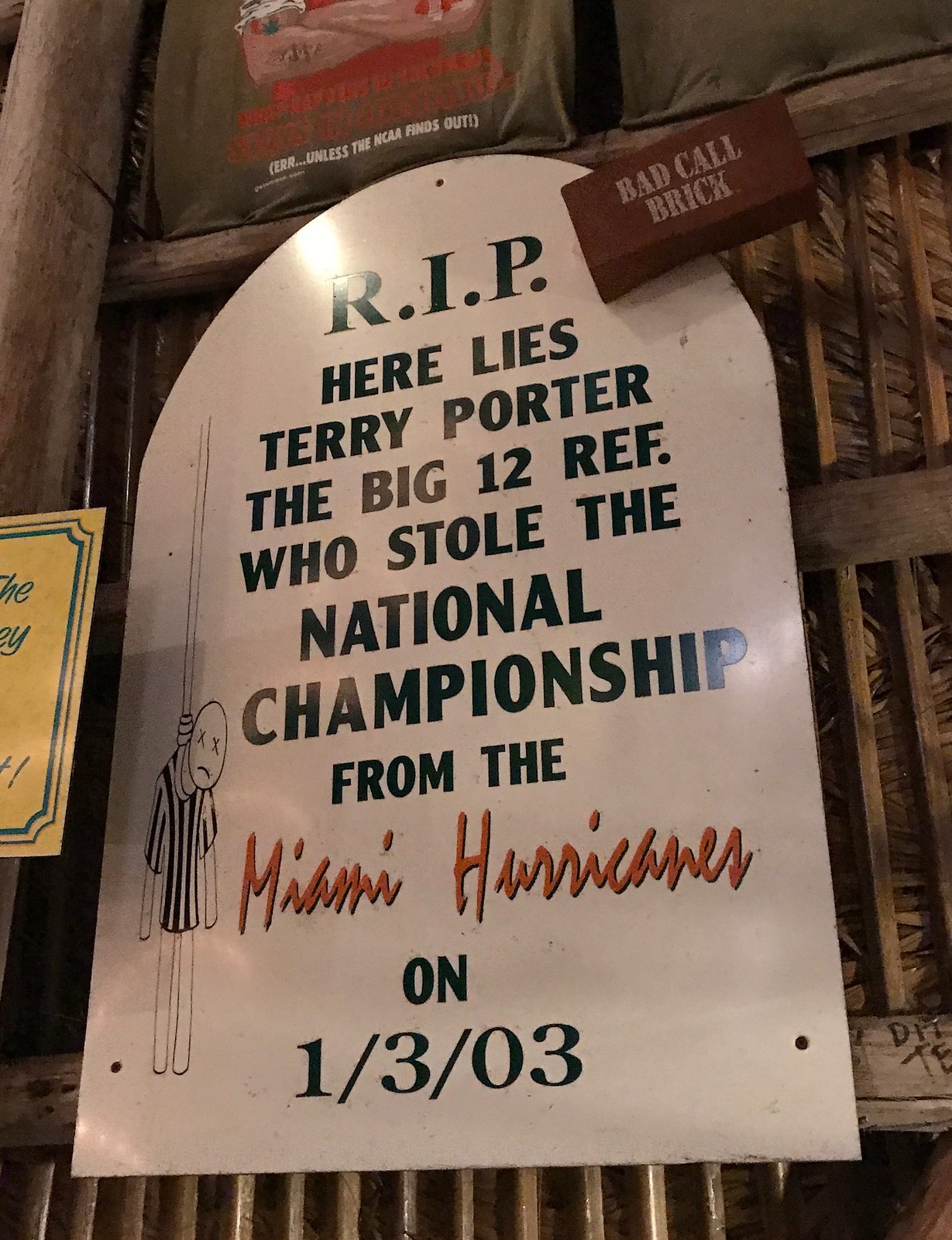This image features a white sign shaped like a tombstone, bolted or hung on a wall that appears to be made of wood and covered with dead palm leaves around the edges. The sign has an arch at the top and a straight bottom. At the top of the sign, bold black letters spell out "R.I.P." Below that, in black text, it reads: "Here lies Terry Porter, the Big 12 ref who stole the national championship from the Miami Hurricanes." The words "Miami Hurricanes" are written in an orange cursive script. Beneath this, the date "1-3-03" is prominently displayed in large black numbers. To the left of the text, there is an illustration of a referee in a black and white striped shirt hanging by a noose. In the upper right corner of the sign, a 3D rectangle has the words "Bad Call Brick" inscribed on it. Another sign in yellow is partially visible on the left side of the image but extends off-screen and is not fully legible.